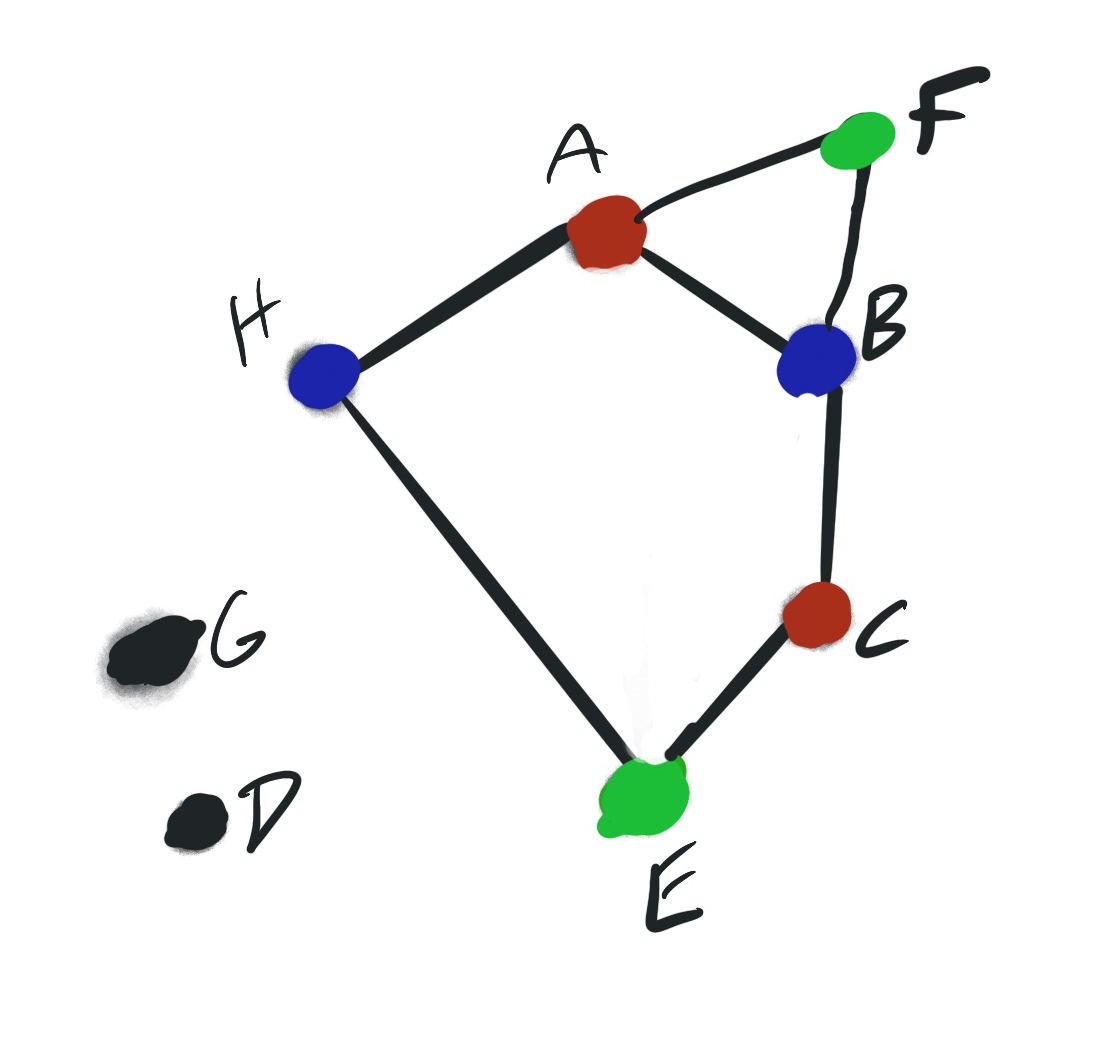This image features a collection of dots and lines set against a white background, initially resembling a graph or a pattern design. In the bottom left corner, there are two imperfectly spherical black dots, reminiscent of painted marks. The upper dot in this pair is labeled with the letter 'G' on its right, and the lower dot is labeled with the letter 'D'.

Moving towards the top right section, a geometric formation emerges. A green dot at the very top right is marked with the letter 'F' to its right. This green dot connects diagonally to a red dot labeled 'A', which lies to its left. Directly below the 'A' dot is a blue dot marked with the letter 'B'. These three dots form a triangular shape, connected by lines.

Furthermore, the red 'A' dot extends to another blue dot labeled 'H', positioned slightly lower and more to the left. This 'H' dot is vertically aligned with a green dot labeled 'E' positioned directly below it. The green 'E' dot is connected by a diagonal line upwards and to the right to a red dot labeled 'C'. The 'C' dot, in turn, connects upwards to the previously mentioned blue dot labeled 'B'.

The intricate arrangement of dots and connections creates a complex and visually engaging pattern, blending artistic design with structured geometry.